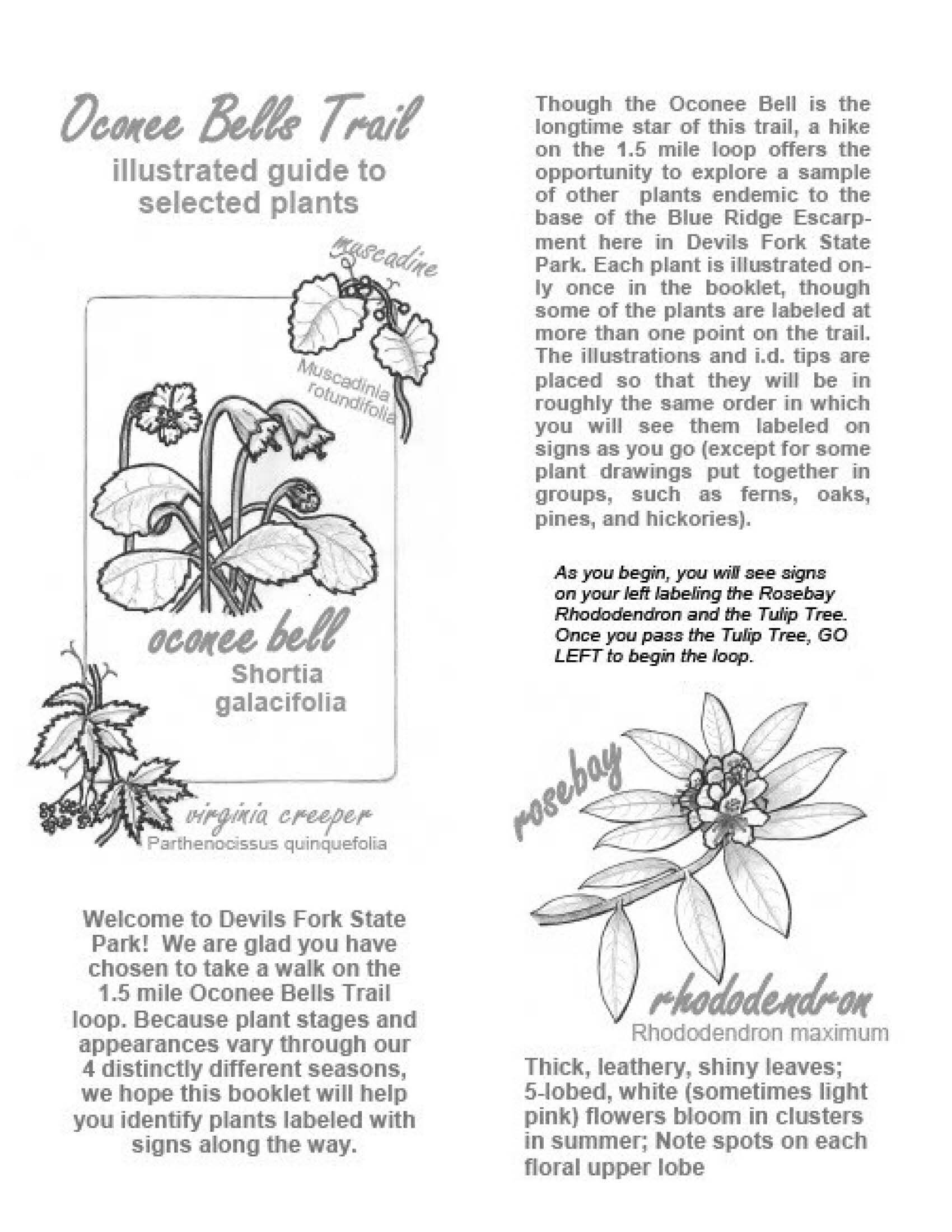The black-and-white image resembles a page from a magazine or an illustrated guide. At the top, it features the title "Oconee Bell's Trail, Illustrated Guide to Selected Plants." The focal point is a detailed drawing of the Oconee Bell (Shortia galacifolia), showcasing its distinctive bell-like flowers, stem, and two leaves on the top right. Also illustrated are Muscadine (Muscadina rotundifolia) with round leaves and Virginia Creeper (Parthenocissus quinquefolia) depicted with small flowers and notched leaves. Another section features the Rose Bay Rhododendron (Rhododendron maximum) with its thick, leathery leaves and five-lobed flowers that bloom in the summer. Ample text throughout the image includes an introductory paragraph that reads, "Welcome to Devil's Fork State Park. We are glad you have chosen to take a walk on the 1.5-mile Oconee Bell's Trail loop." The text elaborates on the trail's seasonal plant variations and emphasizes that a hike on the loop offers the chance to explore other endemic plant species, guiding visitors to match the illustrated plants with the labeled signs along the way.